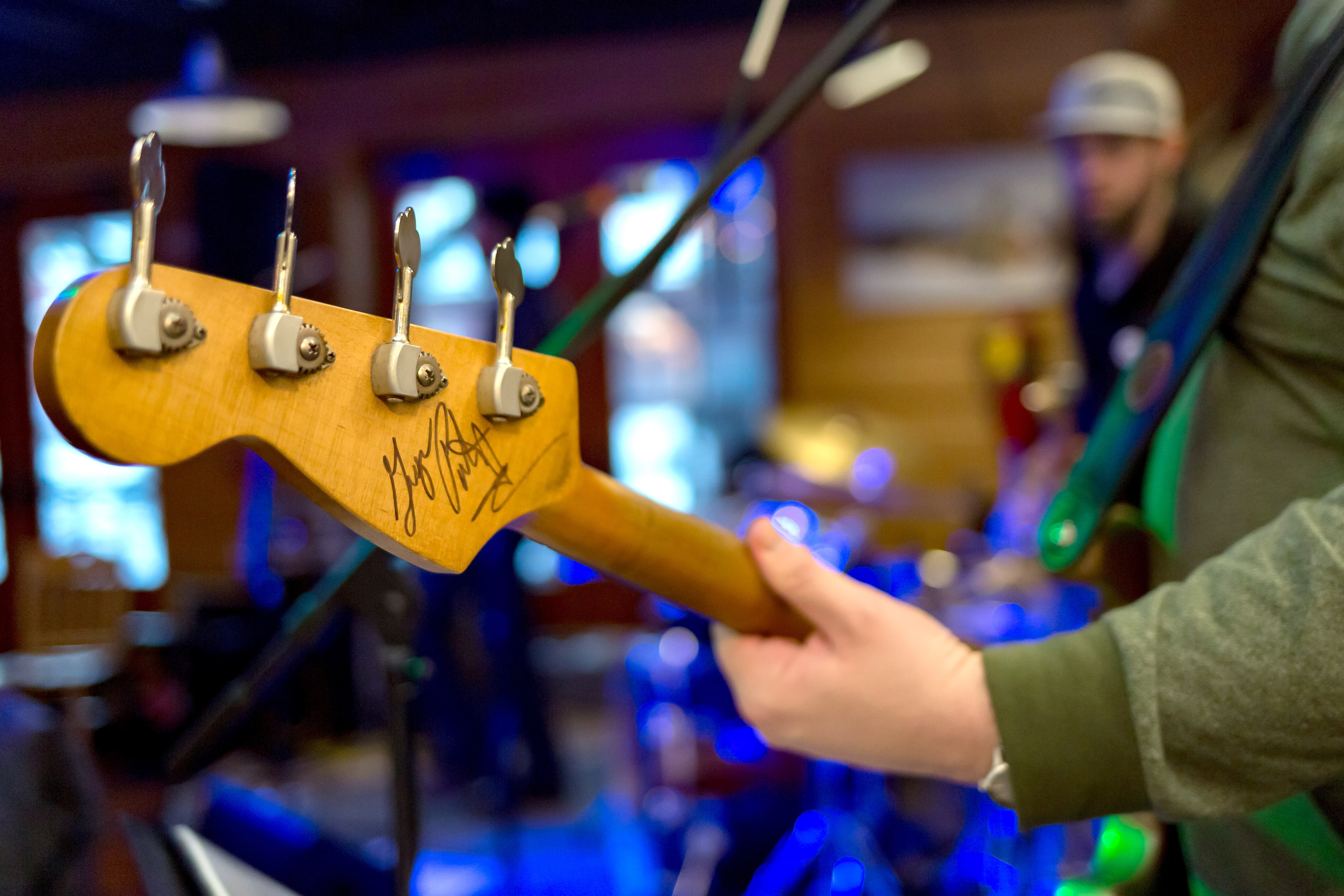This image captures a detailed, intimate moment of a band practice, focusing particularly on a four-string bass guitar from a rear perspective. The focal point is the brown neck of the bass, prominently displaying its tuning pegs and a signature, likely from someone notable, on its backside. The bass is held by a person dressed in a vibrant green long-sleeved shirt or jacket, complemented by a gray-blue strap. A hand is seen strumming the strings, showcasing the personal engagement with the instrument. Surrounding the scene, deep blue chairs or ambient lighting add a contrast, with natural light streaming in from windows that carry a blue tint. In the background, other band members are faintly visible, adding depth and context to the practice session.